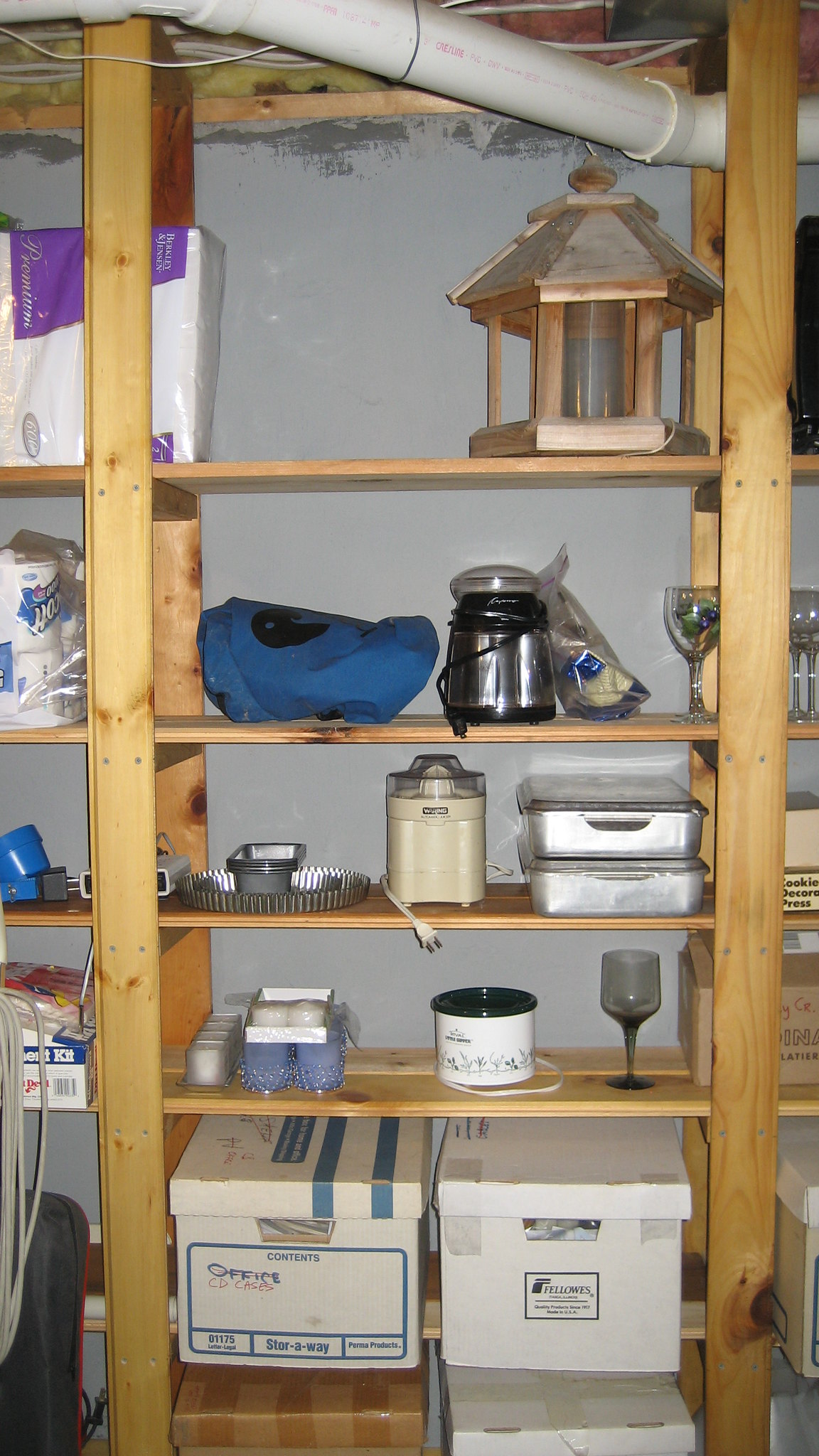This photo captures an organized storage space, likely located in someone's basement rather than a garage, as evidenced by the wooden steps descending from the top of the image. The setting features grey walls with dark grey bricks along the upper portion, adding a textured backdrop to the scene. Dominating the space is a large wooden shelf unit designed for storage, consisting of six rows and three visible columns.

The central column of the shelving unit is fully visible and reveals various stored items. In the first row, there is a wooden birdhouse, a large package of napkins, and something black on the right. The second row houses a package of Scott toilet paper, a piece of blue fabric, a small machine, and what appears to be wine glasses. On the third row, there is a blue plastic item, a metal tin, a beige blender, and two tin trays typically used for carrying food. The fourth row includes another wine glass, a candle, baking tins, and a cardboard box. The fifth row is filled with various cardboard boxes.

The partially-visible side columns contain additional items: the left column is mostly obscured, while the right column shows more storage boxes. The sixth and topmost row appears to contain additional cardboard boxes, one of which is clearly labeled "office." This detailed assemblage suggests a well-organized storage space, utilized for keeping a variety of household items and supplies.